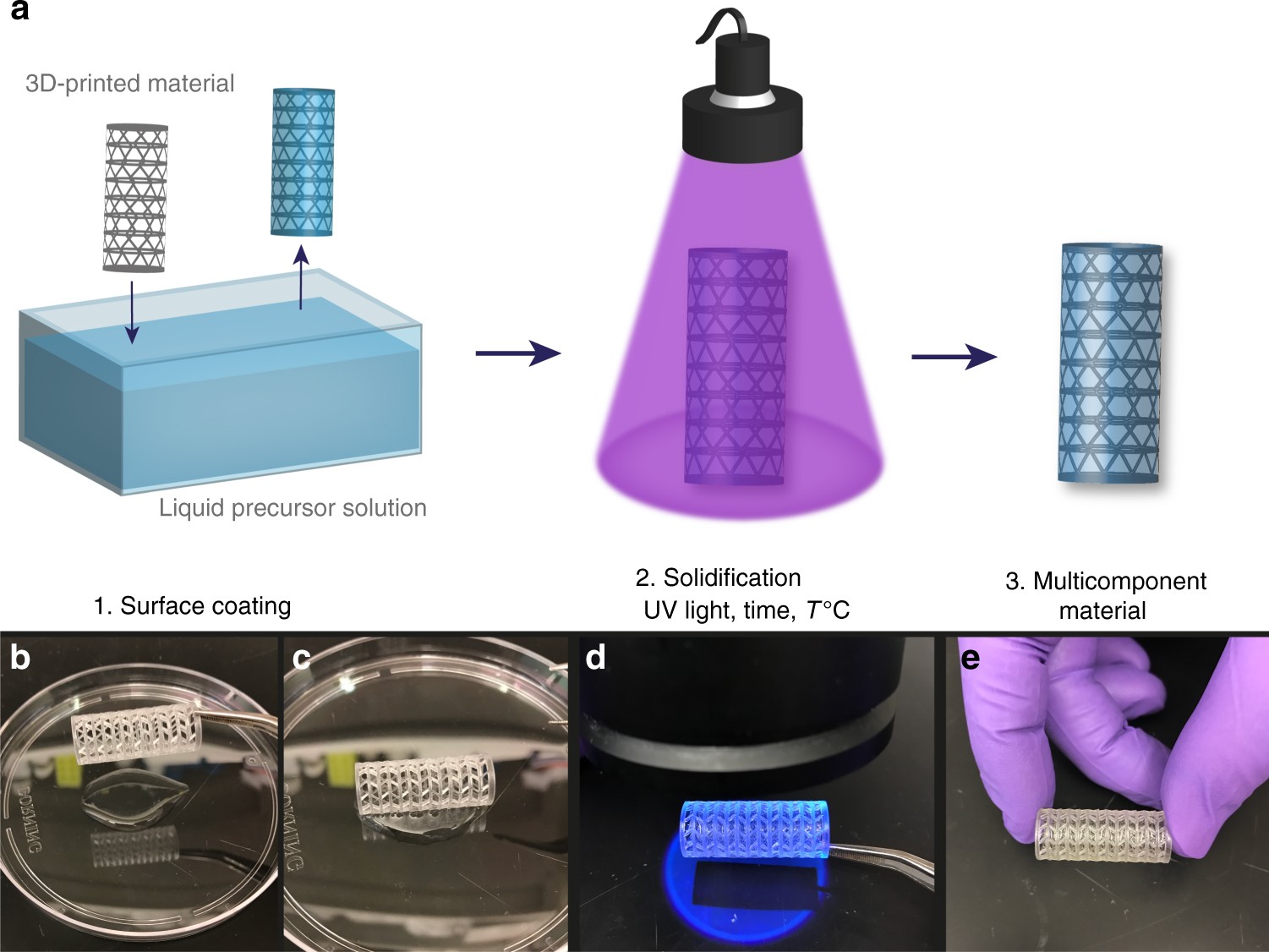The detailed diagram illustrates the process of 3D printing material. At the top left, there's an initial image of a 3D printed material. Below it, a blue rectangular box is flanked by two cylindrical objects. The left cylinder is black and white with triangular patterns, while the right blue cylinder also features triangular patterns. The blue box is labeled "Liquid Precursor Solution," and arrows point right to each cylinder, indicating progression. One arrow leads to a cylindrical object bathed in a purple UV light. Another arrow leads to the blue cylindrical object. The bottom section presents four photographs depicting stages of the process: the first shows a clear circular dish with a white object labeled "First Surface Coating," the second highlights "Solidification under UV light," and the third image shows "Multi-component Material." Additional details mention the UV light operating at 7 degrees centigrade. The step-by-step depiction, combined with the photographs, demonstrates how the 3D printer operates from material preparation to the final product.